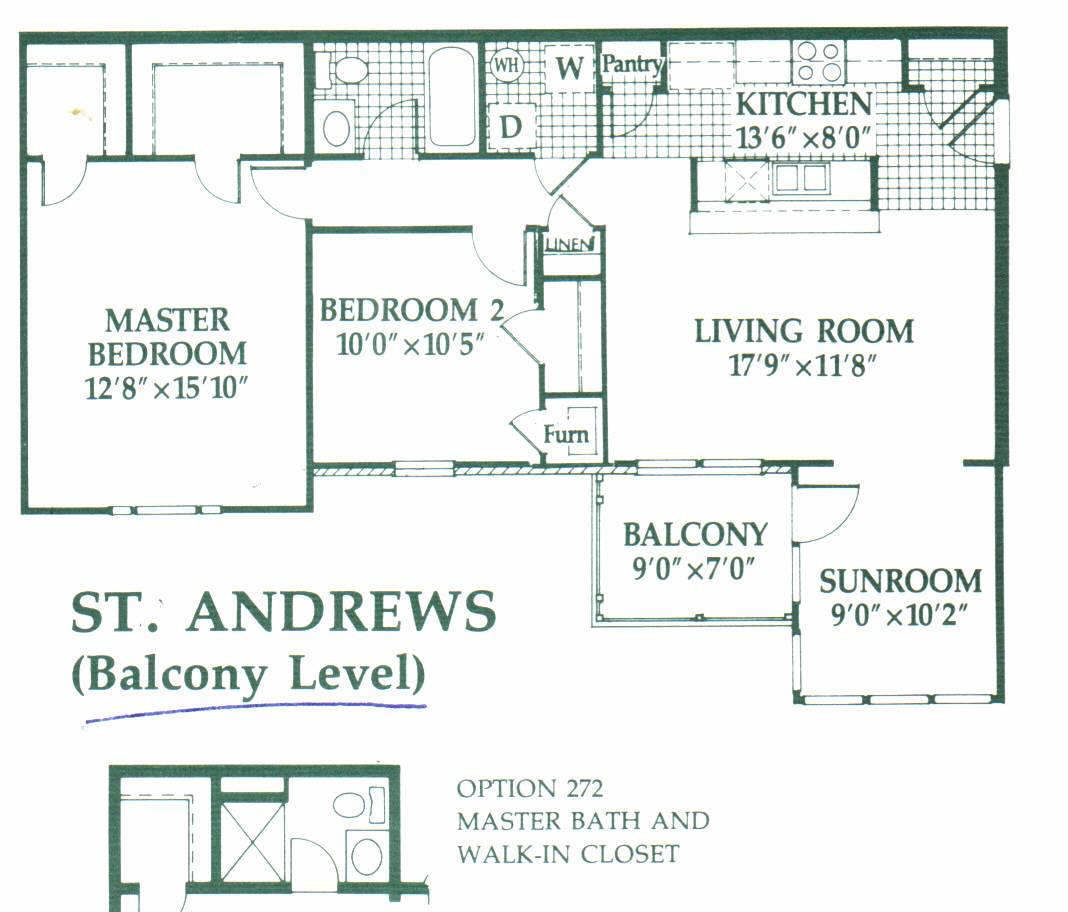This detailed blueprint of St. Andrew's balcony level provides a comprehensive layout of the house. The plan is rendered in green, highlighting various rooms and dimensions. On the left side, the master bedroom measures 12 feet 8 inches by 15 feet 10 inches. Adjacent to it is another bedroom, sized at 10 feet by 10 feet 5 inches, featuring a linen closet and a bathroom nearby. The floor plan also includes a laundry room equipped with a washer and dryer.

The living room, which measures 17 feet 9 inches by 11 feet 8 inches, is centrally located. Connected to the living room is the kitchen, measuring 13 feet 6 inches by 8 feet, which includes a pantry for additional storage. Off the living room is a sunroom that is 9 feet by 10 feet 2 inches, providing ample natural light. The sunroom opens to a balcony, which is 9 feet by 7 feet, ideal for outdoor relaxation.

Moreover, this St. Andrew's balcony level blueprint includes optional features labeled as Option 272. This option offers an extended master bath and a walk-in closet for enhanced convenience and luxury in the master suite.